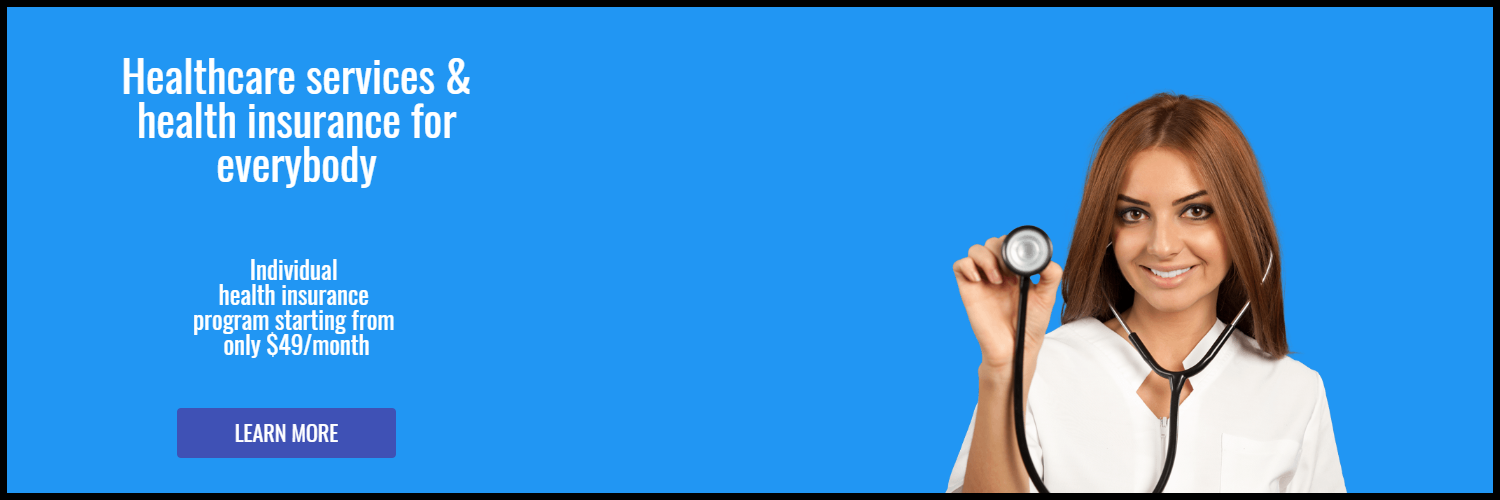This image appears to be a professional advertisement for health care services and health insurance, featuring a clear and vibrant design. The main background is a large blue rectangle framed by a black border. Positioned to the left side in bold, easy-to-read white font, the text reads: "Health Care Services & Health Insurance for Everybody." Below this, the text continues with: "Individual Health Insurance Programs starting from only $49 a month." 

Additionally, there is a dark blue call-to-action button with the words "Learn More" prominently displayed in white. 

On the right side of the image, a smiling woman with brown hair is featured. She has dark brown eyebrows, wears dark-colored eyeshadow, and appears to have brown or dark eyes. She is dressed in a white scrub top and has a stethoscope around her neck, with the earpieces in her ears and the chest piece held up in her hand. The stethoscope is black and silver.

The entire image is of high quality, free from blurring or pixelation, and the fonts are large and bold for easy readability. While the design is slightly amateur-looking, it effectively communicates its message.